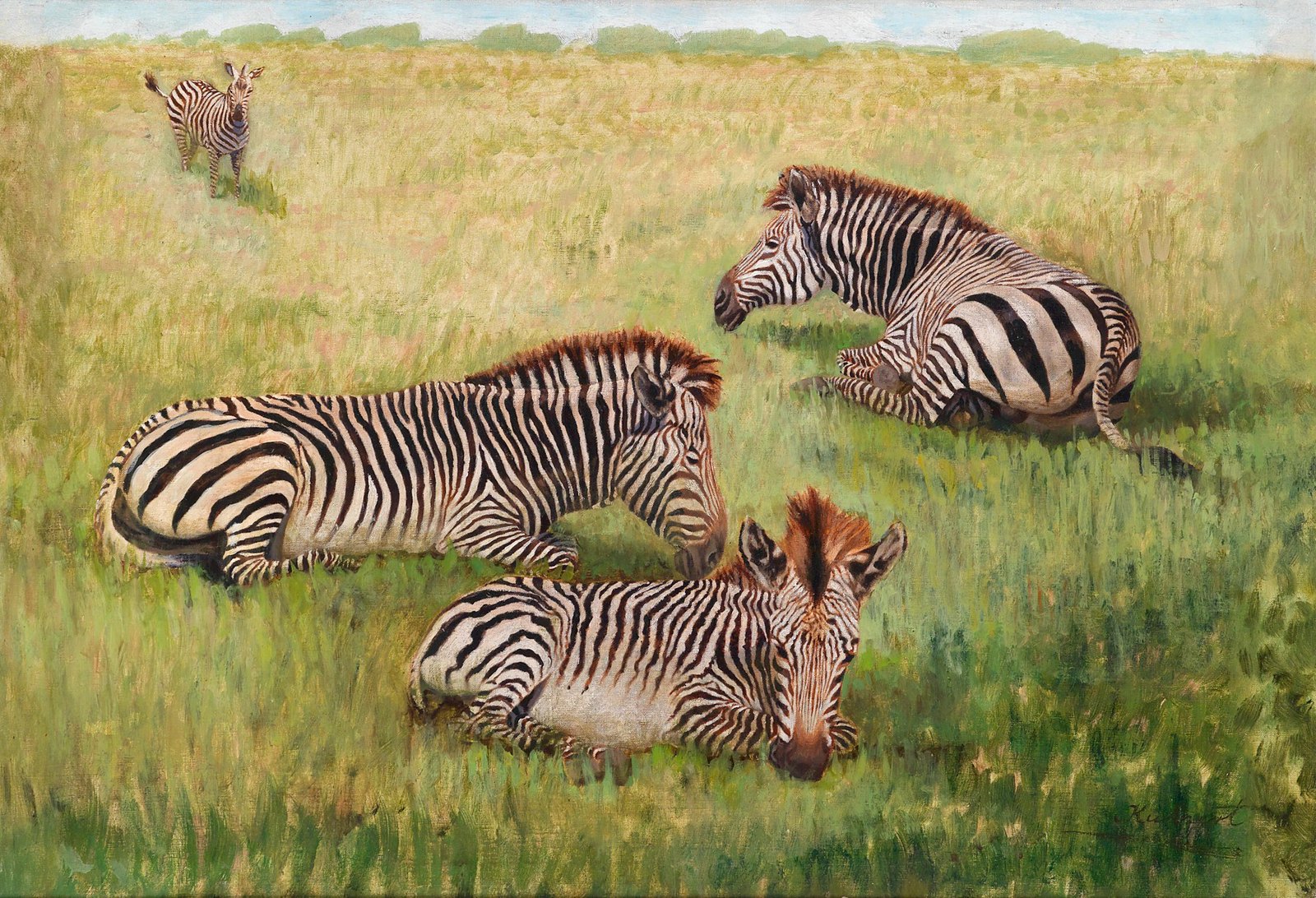The image is a detailed oil painting of four zebras situated in a serene savanna setting. The composition includes a mix of green and yellow grasses, executed with soft, splotchy strokes typical of oil painting. In contrast, the zebras are rendered with precise details, highlighting their black and white stripes.

Three zebras are lying down, resting. One of these zebras, positioned centrally, gazes directly at the viewer. To its left, another zebra lies down, its head turned to profile. The third zebra, located in the upper right corner, is also lying down, presenting a partial side and back profile. The fourth zebra stands in the upper left corner, observing the others.

The field transitions in color from a bright green at the bottom to a yellowish-green as it extends upward. Treetops and a sliver of a cloudless, light blue sky frame the scene at the top, though both are out of focus.

A signature in a gray or black font is present in the lower right corner, featuring discernable letters such as "K," "U," and "T," underscored by a line, confirming the work as a painting and adding an element of authenticity.